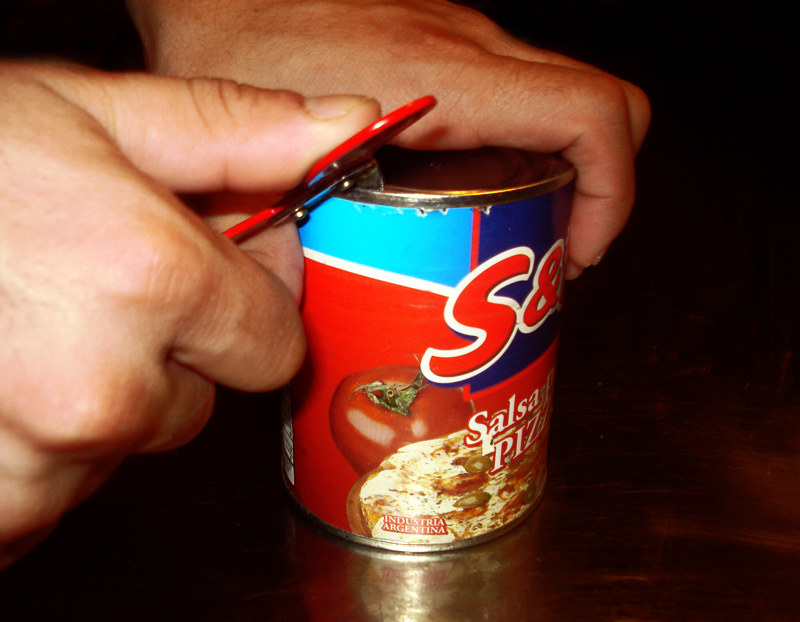A close-up image captures a pair of hands engaged in opening a can. The left hand firmly holds the can, while the right hand wields a can opener with a red handle, pressing it into the silver top of the can to pry it open. Surrounding the top edge of the can, there is a distinct silver rim. Toward the right edge of the image, there is a light blue background intersected by a vertical white strip.

The front label of the can prominently features a large "S" and an ampersand ("&") set against a sizeable blue square. To the right of this, the label has a vivid red section illustrating a ripe tomato accompanied by lush green leaves. Additionally, the label displays an appetizing image of a salsa pizza, topped with slices of pepperoni, jalapeños, and melted cheese. Written on this section is the word "Argentina," indicating the product's origin. Light reflections on the can add a gleaming effect, contrasting against the black background that forms the base of the image.